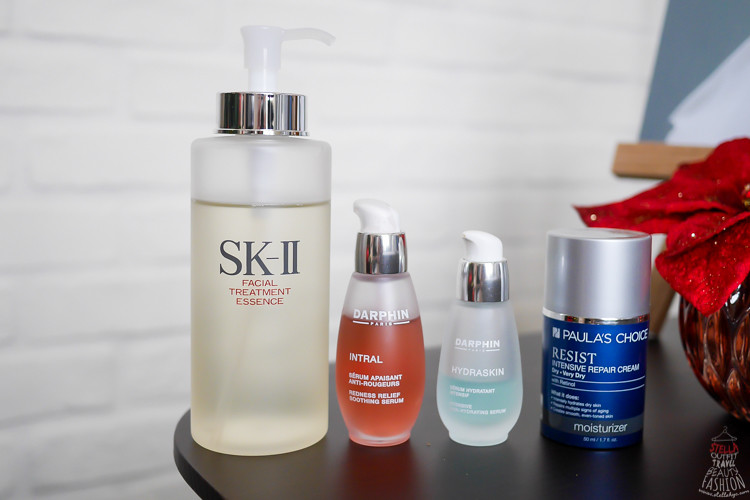The image features a collection of four diverse beauty products neatly arranged on a round wooden table.  

1. The first and most prominent product is presented in a large, transparent glass bottle topped with a metal lid. It features a sleek lotion dispenser and is labeled with "SK-II" in crisp black lettering. Below the main label, in vibrant red text, the product is identified as "Facial Treatment Essence."

2. The second product stands at approximately two-thirds the height and diameter of the first. Encased in an elegant frosted glass container with a metal cap and lotion dispenser, it bears the brand name "DARPHIN." Below this, the label reads "INTRAL" in stark white text, with the liquid inside revealing a subtle reddish hue.

3. Positioned next is a similarly shaped yet slightly smaller container, also made of frosted glass and topped with an aluminum cap and a white lotion dispenser. This product is also from "DARPHIN" and is marked with "HYDROSKIN" in white letters.

4. The final product diverges in design, boasting a cylindrical blue container with a silver cap. Its bold white text identifies it as "PAULA'S CHOICE, RESIST, INTENSIVE REPAIR CREAM," accompanied by additional smaller writing below.

This carefully curated arrangement showcases the diverse range of beauty products, each distinguished by its unique design and packaging.